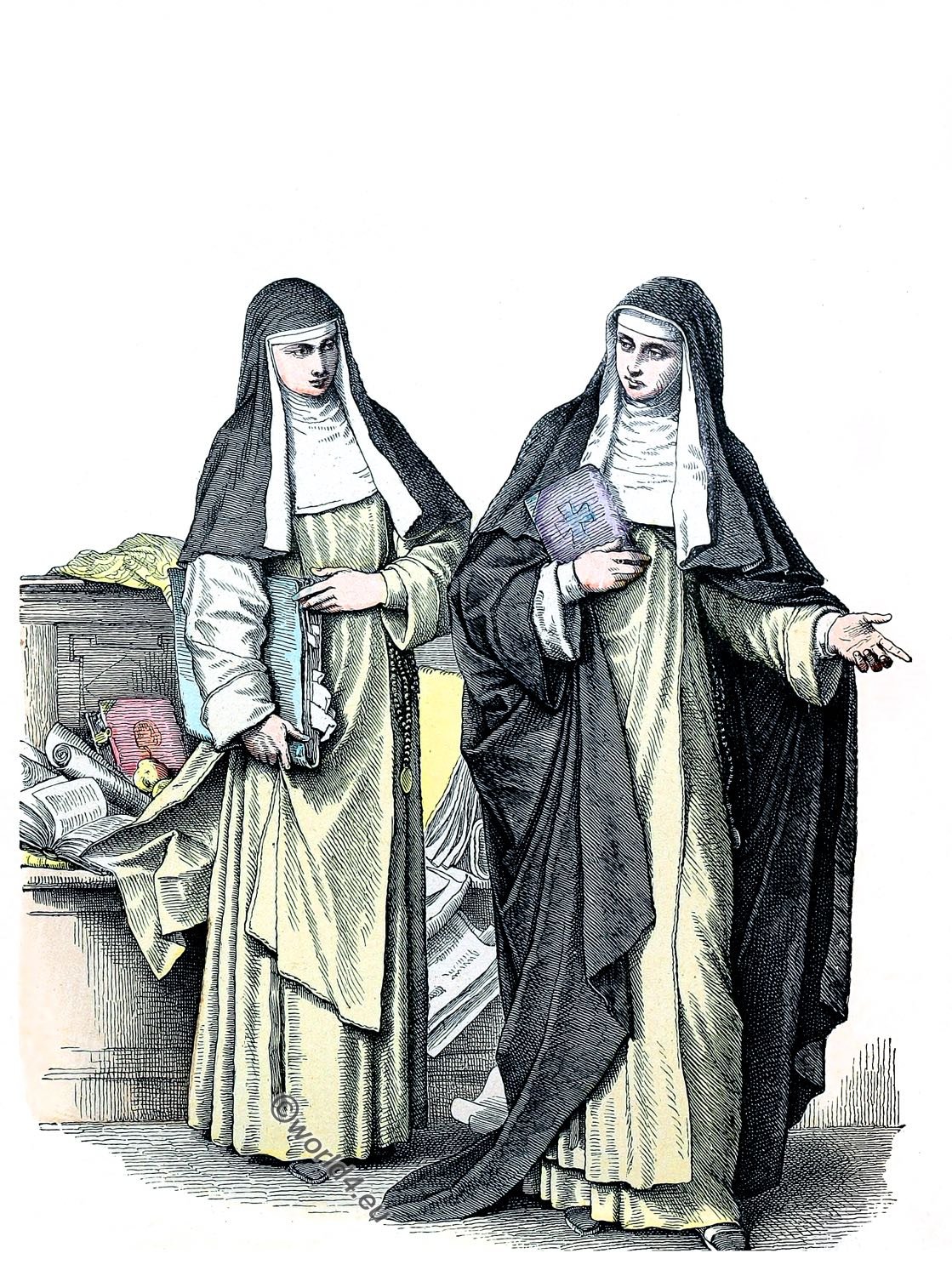This detailed image is a drawing of two nuns dressed in long, flowing gowns and head coverings that resemble traditional habits. Both their heads and bodies are completely covered, including their feet. They appear to be wearing black shawls or cloaks over green dresses or robes, and a chain hangs down around hip level. 

The nun in the foreground, positioned on the left, is holding a manuscript in her right hand, tucked down to her side and stabilized with her left hand across her waist. The nun on the right is pointing and giving directions with her left hand while holding a small black book with a blue cross — likely a Bible — close to her chest in her right hand. Behind them is a bench with various items on it, including an open box containing papers, books, a scrolled-up paper, and potentially a red book. A yellow garment is draped across the bench. The background of the image is white, and a watermark at the bottom reads "copyright world 4.eu."